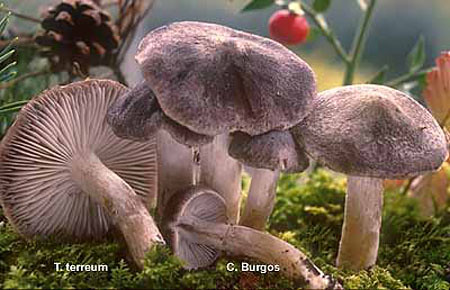The image features a cluster of mature wild mushrooms with grayish light brown caps and wide, somewhat eroded white stems, situated in a small field-like area with brownish soil interspersed with patches of green. Several of the mushrooms have toppled over, revealing the interior caps, though their stems remain rooted in the ground. In the background, a tomato plant with a single red tomato hangs on the right side, and a pine cone is visible on the ground to the left. The setting appears to be a natural, forest-like environment, with additional elements including some grass and scattered leaves. The mushrooms, numbering at least five, dominate the foreground, while the other elements provide contextual details around them.